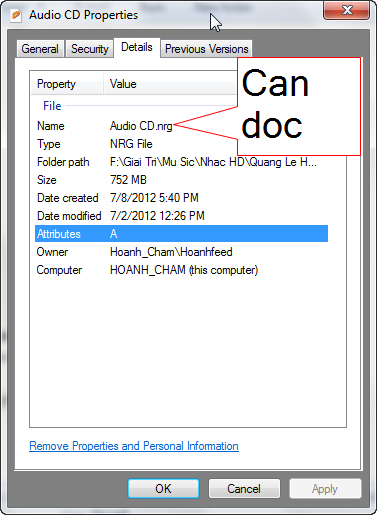This image is a detailed screenshot taken from a Windows Vista computer, capturing the "Audio CD Properties" dialog box. The familiar mouse cursor is visible, suggesting it is a computer-generated image rather than a mobile screenshot. At the top, the dialog title "Audio CD Properties" is displayed, along with the standard window controls, including a red X button in the upper right corner.

The interface features four tabs: General, Security, Details (which is currently active), and Previous Versions. Under the Details tab, a table categorizes information into "Property" and "Value." The properties listed include Name (audio CD.NRG), Type, Folder Path, Size (752 MB), Date Created (7/8/2012 at 5:40 PM), Date Modified, Attributes, Owner, and Computer. Additionally, there is a link to remove properties and personal information.

At the bottom of the dialog box, three buttons are present: OK (highlighted), Cancel, and Apply (grayed out, or disabled). The colors in the screenshot predominantly feature shades of red, white, gray, black, and light blue. Overall, the screenshot focuses solely on this Windows Vista dialog box, occupying the entire image without any additional objects in view.